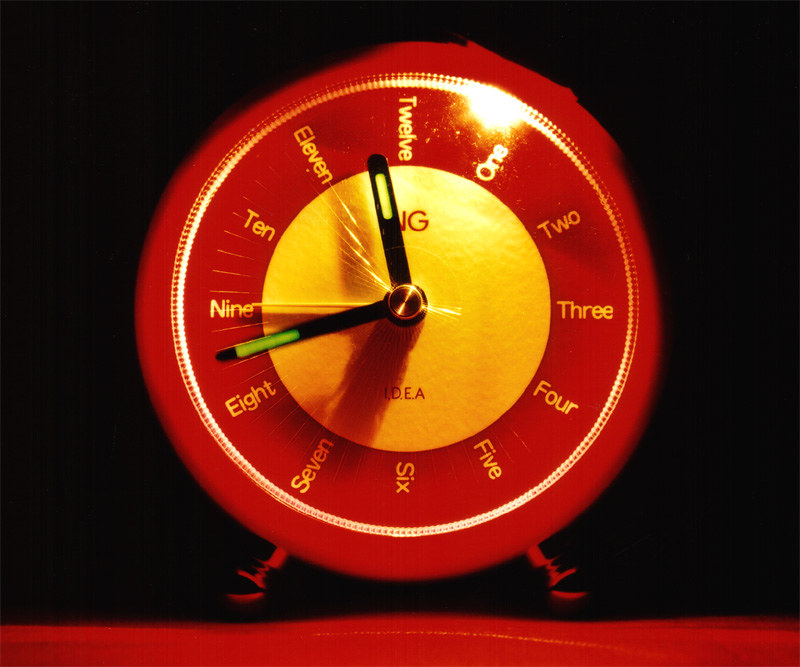The image is a piece of detailed digital artwork featuring a vivid, fire engine red circular clock set against a dark, black background. The bottom portion of the background is bordered by a somewhat uneven red strip, possibly representing a table surface with red legs. The clock, seemingly mounted on a wall, has a striking design with a large, flat gold center surrounded by concentric circles. The clock numbers are written out as words rather than numerals, with “12” at the top followed sequentially by “1,” “2,” “3,” and so on, enhancing its unique character. Encircling the clock face is an outline defined by white and yellow lines. The clock's black minute hand features a green rectangle at its tip, the black hour hand has a yellow top, and the slender second hand is yellow. The time displayed on the clock is 11:43.